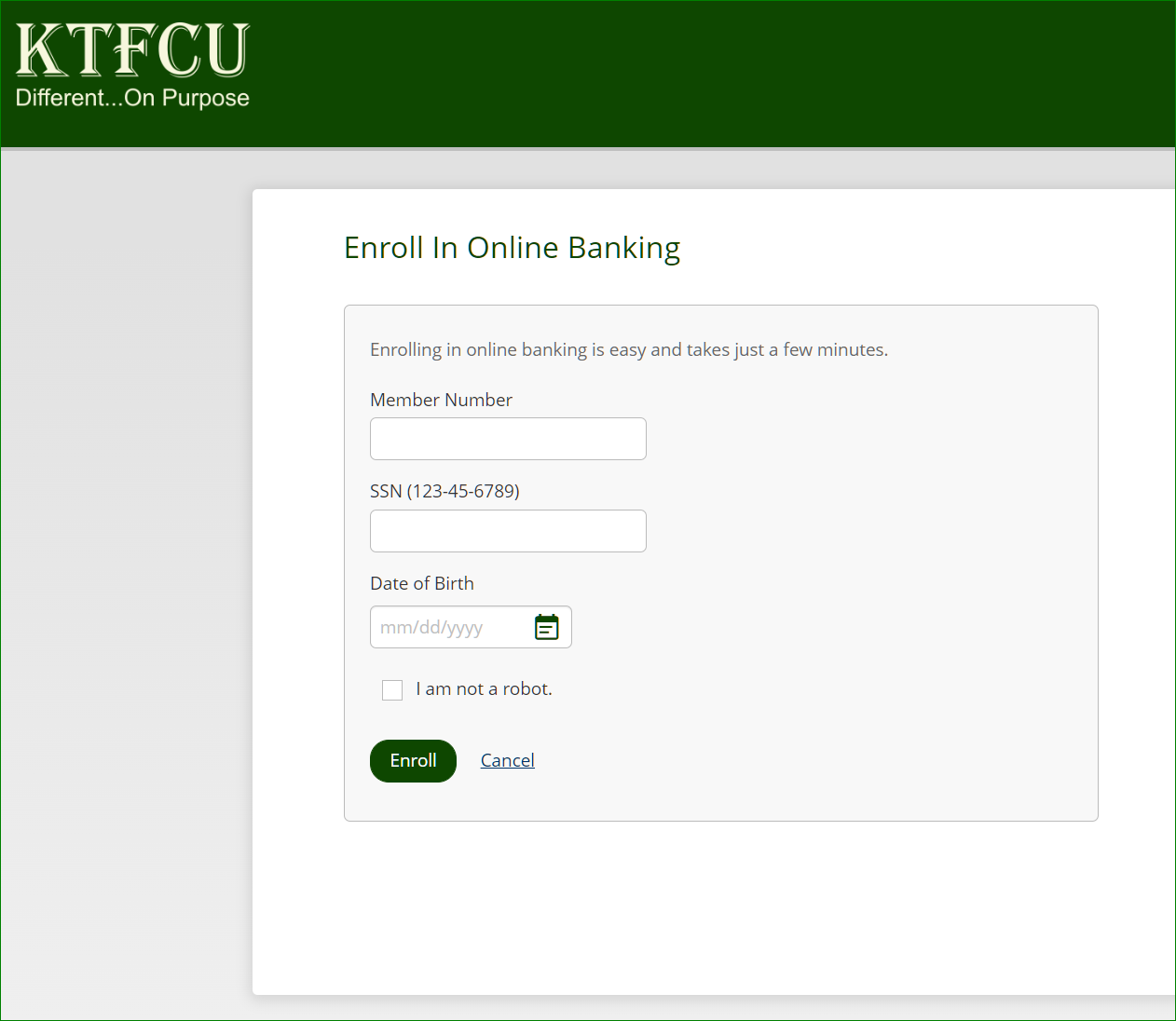The image depicts a screenshot from a website, specifically from the page of a financial institution. At the top left corner, a green rectangle features the acronym "KTFCU" written in elegant, almost calligraphic capital letters, in a cream color. Below it, the tagline "Different... on Purpose" is also visible in the same cream-colored calligraphy.

Towards the lower right-hand corner, there is a white rectangular section over a gray background. The top part of this white rectangle contains a green-colored prompt that reads, "Enroll in Online Banking." Below this prompt in the gray area, there is text in greyish tones that states, "Enrolling in online banking is easy and takes just a few minutes."

The form provides fields for user input, including "Member Number" and "SS Number," with an example format for a Social Security Number. Additionally, there is a field for "Date of Birth," which shows the format "MM-DD-YYYY" beside a calendar icon. At the bottom of the form, there is a checkbox labeled "I am not a robot," followed by an "Enroll" button and a "Cancel" button, allowing users to proceed with or abort the enrollment process.